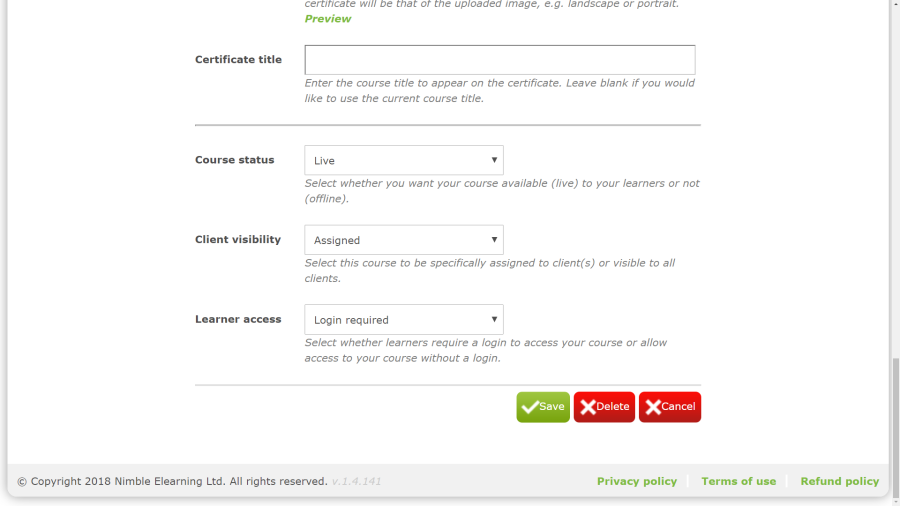This image is a detailed screenshot of the lower right-hand corner of a website interface. The very bottom of the image features a narrow light gray border that contrasts with the white page background. On the lower left-hand corner, the text "© 2018 Nimble eLearnings Ltd. All rights reserved." is elegantly displayed in gray font.

In the lower right corner, green-font links are clearly visible, including "Privacy Policy," "Terms of Use," and "Refund Policy."

The primary content of the image focuses on a form. On the left side, appearing in gray font, the label "Certificate Title" is prominent. Directly below, there is a rectangular input field with placeholder text instructing users: "Enter the course title to appear on the certificate. Leave blank if you would like to use the current course title."

Moving further down, "Course Status" is labeled on the left, accompanied by a drop-down menu currently displaying the option "Live." Beneath this, a description states: "Select whether you want your course available live to your learners or not (Offline)."

Next, the section "Client Visibility" has its own drop-down menu, with the option "Assigned" currently selected. Below it, guidance reads: "Select this course to be specifically assigned to clients or visible to all clients."

The final section labeled "Learner Access" also features a drop-down menu, showing "Login Required." The description beneath advises: "Select whether learners require a login to access your course or allow access to your course without a login."

At the bottom of the form, three action buttons are aligned horizontally. The first is a green button with white text and a checkmark icon that says "Save." Next to it, a red button with white text and an X icon says "Delete." The third button, also red with white text and an X icon, reads "Cancel."